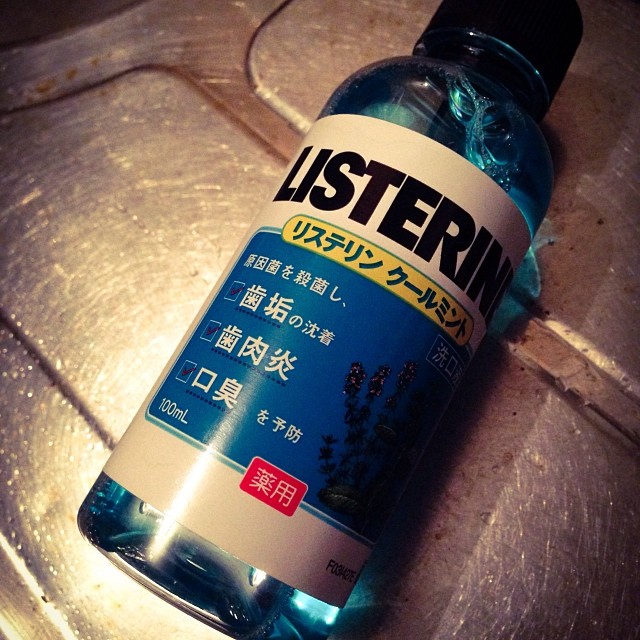The image depicts a bottle of Listerine laying on its side on a scratched, silver-like metallic surface, which could be a sink, a medical tray, or a counter. The bottle is filled with a typical aqua blue liquid and sealed with a black cap. The prominent white label on the bottle features the Listerine brand name in bold black letters. Below this label, a small yellow banner displays Oriental characters, followed by a blue rectangular section containing three bullet points marked by check marks, each accompanied by more Oriental text. Near the bottom of the blue rectangle, the text indicates the bottle's capacity as 100 milliliters. Additionally, there is a small red rectangle at the base of the blue section with Asian characters, further detailing the product.